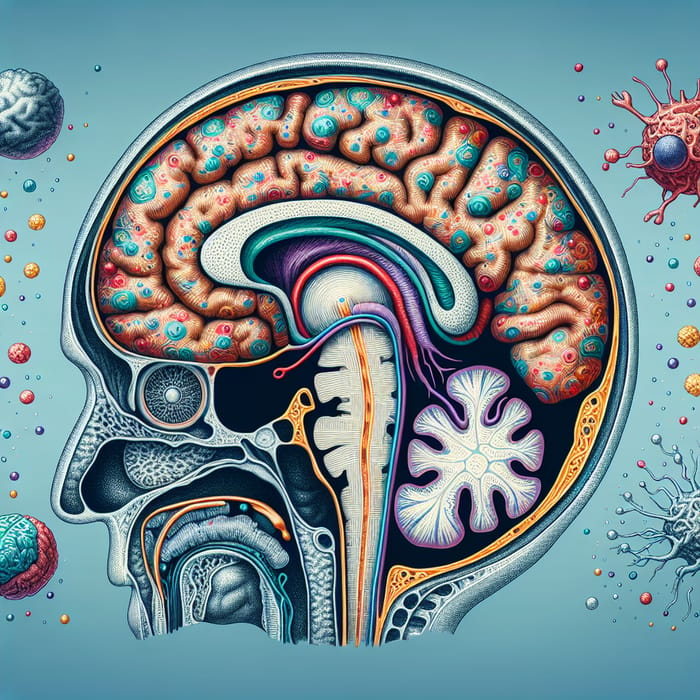The image is a detailed cutaway view of a human skull, revealing the complex internal structures of the brain. The brain itself is depicted in a beige or light orange-brown hue, marked with round blue and red areas, possibly representing different functional zones or anatomical features. Central to the brain's structure, the brain stem appears prominently, extending downward in a yellow line symbolizing the spinal cord, cushioned by gray matter. In the lower right section of the brain, a purple, leafy-looking structure is visible, adding to the intricate depiction. Towards the bottom left quadrant of the image, the nasal cavities, eye socket, and parts of the tongue are illustrated in varying shades of blue, lending a color-coded clarity to the anatomical diagram.

Encircling the main image of the skull, the background is a light blue-gray, populated with numerous spherical blobs of varying colors, intended to represent cellular structures or microscopic entities. These blobs, which include shades of yellow, red, purple, blue, and green, appear to float around the skull. Some of these spheres possess tentacle-like extensions, particularly a red blob in the upper right and a blue-gray one in the lower right, possibly suggesting different types of cells or microorganisms. The entire composition presents a vivid, multi-colored exploration of human anatomy against a serene, light blue background.